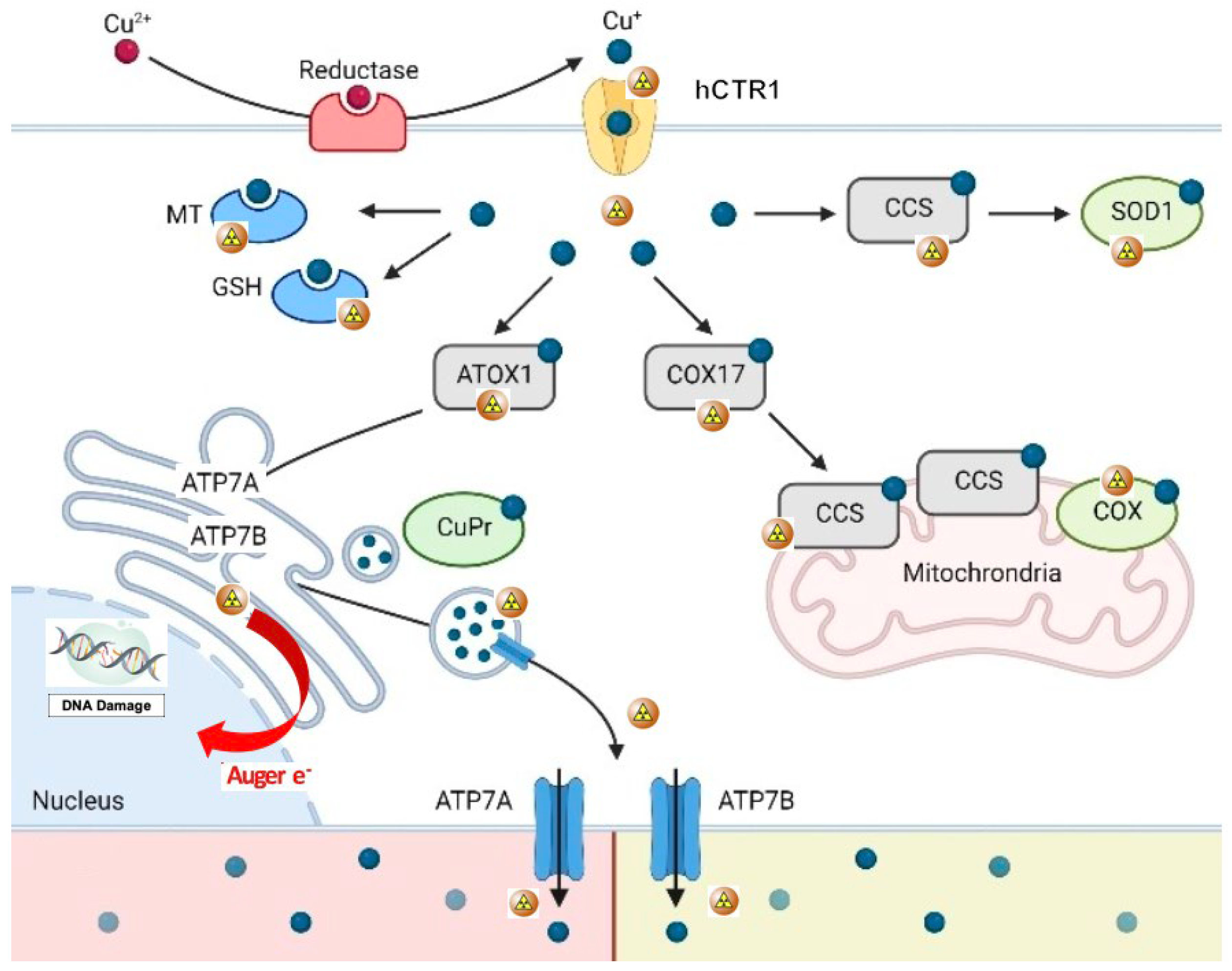This is an informational diagram on a white background illustrating the cellular transport and effects of copper ions, specifically Cu2+ and Cu+. At the top left, a silver dot labeled "Cu2+" connects via a black line to a red dot surrounded by a pink layer, labeled "Reductase." From there, a black arrow leads to a blue dot labeled "Cu+." Below this, there's a yellow encapsulated blue dot labeled "HCTR1." Additionally, two blue dots surrounded by blue and marked with radioactive symbols are labeled "MT" and "GSH." Further along, blue dots within gray triangles are labeled "ATOX1" and "COX17." Another blue dot, off to the side, labeled "CCS," and a green oval-shaped dot, labeled "SOD1," are connected to the ATOX1 pathway.

The diagram also features blue squiggly lines at the bottom left, showing branches leading to "ATP7A" and "ATP7B." These lines branch out to a green oval labeled "CUPR," indicating copper transport pathways. A red arrow depicts how copper ions enter the nucleus, causing DNA damage. Lastly, the "COX17" label leads to two light gray boxes labeled "CCS" and a green oval labeled "COX," all integrated within a purple kidney bean-shaped mitochondrion. The diagram explains the complex interactions of copper ions within cellular structures, including the mitochondria on the right and the nucleus on the left.